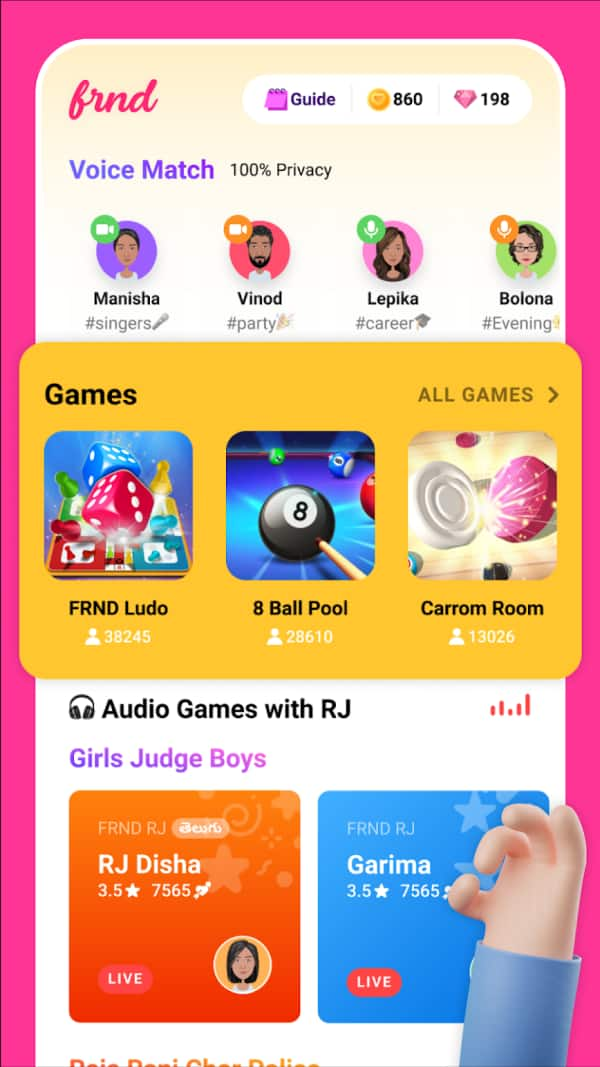This image showcases a mobile app interface with a pink-themed design. The photo is in portrait orientation, resembling the shape of a cell phone with a pink border surrounding the screen. The internal app display is also pink with rounded rectangular edges.

At the top of the screen, there are purplish-pink letters forming the partially visible text 'FR' and 'D,' likely abbreviating the app name to something akin to "Friend." Below this title, there is a prominent white, oval-shaped box divided into three segments. These segments read: "Guide," followed by a display of 860 coins and a diamond icon next to the number 198. Another section reads "Voice Match" in blue text, emphasizing "100% Privacy."

The middle section of the screen displays four avatars, consisting of one man and three women. Beneath these avatars is a yellow rectangular box oriented in landscape that promotes gaming options with the word "Games" and suggestions for three different games.

Towards the bottom portion of the interface, a header labeled "Audio Games with RJ" appears, followed by a subheading "Girls Judge Boys," and two clickable thumbnail images. The first thumbnail is labeled "RJ Desha," and the second one is marked "Guram." On the right side of this section, there is an icon depicting a hand extending out from a sleeve with a blue cuff, adding an interactive element to the app's design.